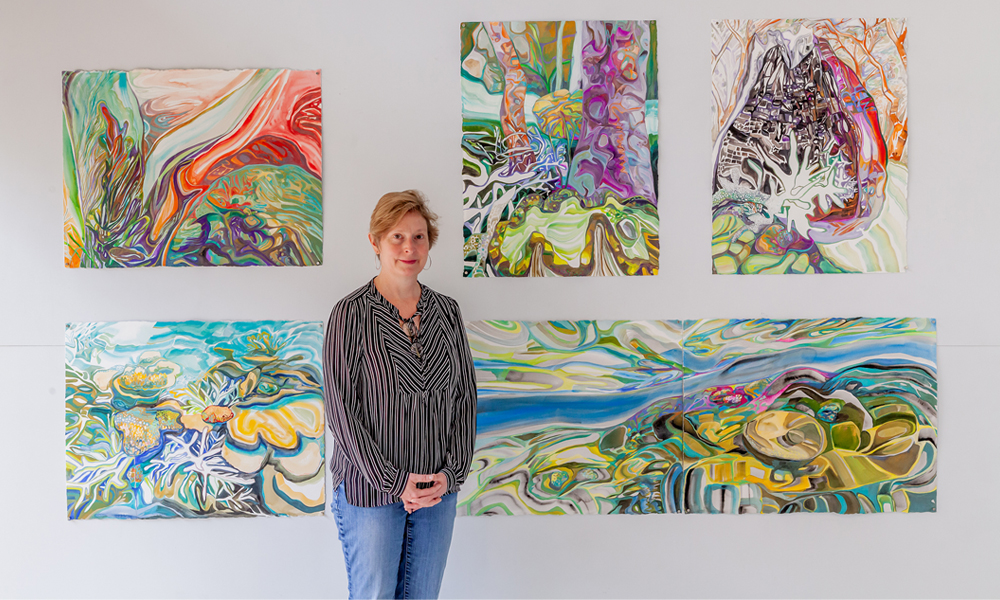A woman with short blondish-brown hair, wearing a black-and-white striped blouse, blue jeans, hoop earrings, and prescription glasses hanging from the neck of her top, stands casually with her fingers interlocked in front of her. She is posing in front of a wall adorned with five vibrant paintings. The paintings feature abstract, amorphous designs reminiscent of neo-Van Gogh and colorful abstract expressionism styles. The upper three paintings are all more portrait-shaped, filled with psychedelic colors and organic shapes, depicting what looks like underwater imagery or the interior of the human body. The lower two paintings include one large, rectangular piece that is three or four times wider than it is tall and a square-like painting, both showcasing similar organic and colorful abstract designs. The overall aesthetic of the artwork is vibrant, with reds, greens, and yellows creating a mesmerizing display behind the woman.